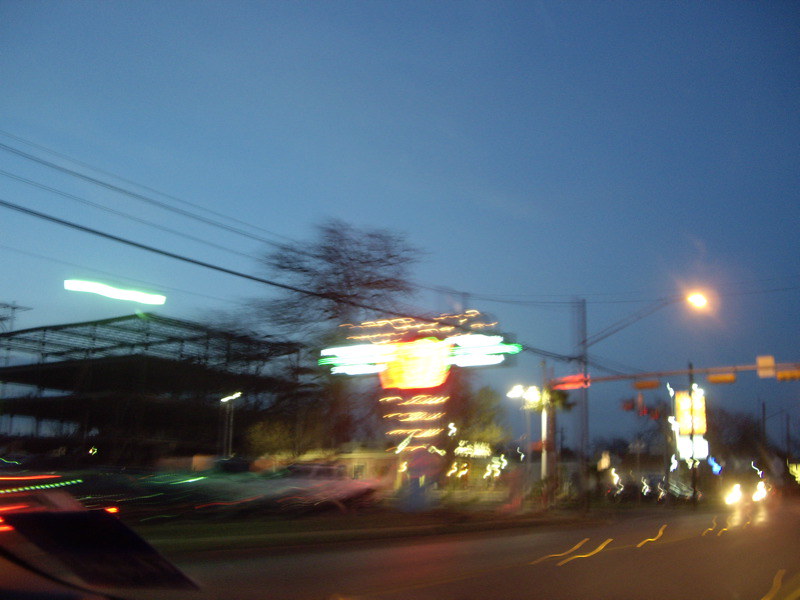This photograph, taken at night, captures a blurry street scene seemingly shot from inside a vehicle. In the foreground, a bright, illuminated sign dominates the image. The sign features vibrant green and yellow lighting, with the main design resembling a yellow sun flanked by green cloud-like shapes. Above and below this central motif, yellow illuminated writing is somewhat discernable. This sign stands in front of an incomplete structure, revealing a steel frame and floor plates, though no walls or further details are visible.

Ambient lighting reflects off the glass, indicating the photograph was likely taken from within a car. Approaching head-on, the headlights of another vehicle pierce through the darkness, adding to the reflective interplay of red and green lights on the left side of the image. These reflections contribute to the overall sense of motion and depth.

A silver pole stretches across the roadway, supporting a horizontal array of three yellow stoplights, hinting that the vehicle the photograph was taken from might be nearing an intersection. The asphalt road lies beneath, barely visible under the layers of blurring and light reflection. Additional cars seem to line the side of the road, but the blur renders further identification impossible. The combined elements of urban infrastructure, artificial light, and vehicular motion create a vivid, if indistinct, portrayal of a nighttime urban environment in transition.